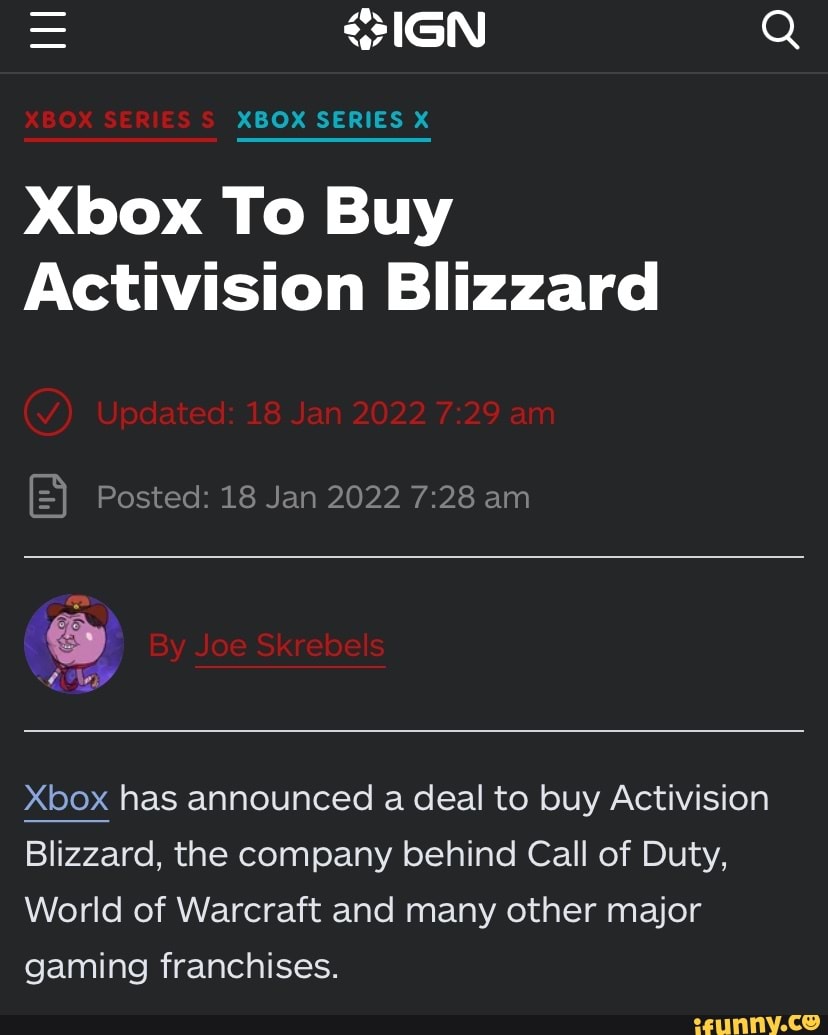The image features a predominantly black screen with text in various colors. In the upper left corner, there are three stacked bars. At the center, the logo "IGN" appears; however, it initially resembles "OIGN" due to a cross-like symbol intersecting the "I". To the right of this logo is an icon of a magnifying glass. Underneath these elements, a horizontal line separates the top portion from the main text.

The main text begins with "Xbox Series S" in red, underlined, followed by "Xbox Series X" in blue, also underlined. Below this, in white text, it states "Xbox to buy Activision Blizzard," accompanied by a red circled checkmark. Next to this, it reads "updated 18 Jan 2022 7:29 AM" in red text. Proceeding further, there is an icon of a piece of paper with lines, indicating a posted update at "18 Jan 2022 7:28 AM" in light gray text.

Another white horizontal line introduces the author section, where "by Joe Skrebels" (with "Joe" and "Skrebels" underlined in red) appears. The word "by" is in red as well. Following another white horizontal line, the text in light blue underlined says, "Xbox has announced a deal to buy Activision Blizzard, the company behind Call of Duty, World of Warcraft, and many other major gaming franchises."

In the bottom right corner, the watermark "ifunny.co" is displayed in yellow.